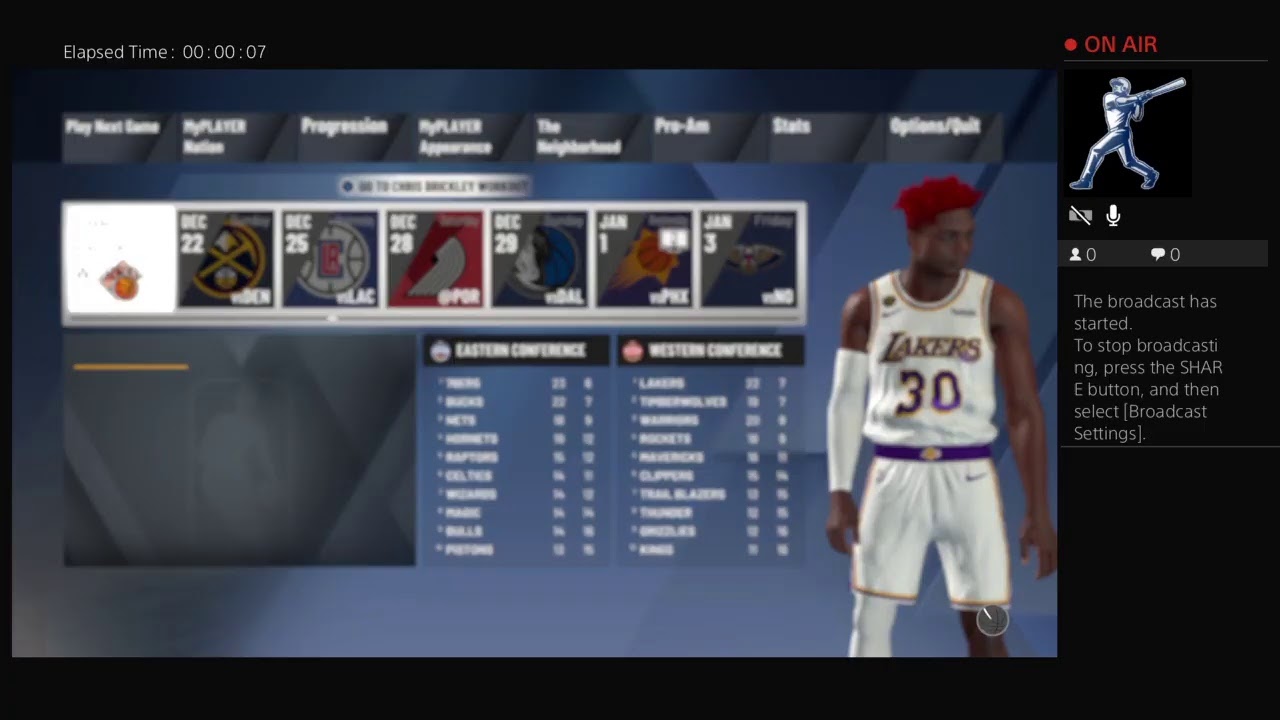The screenshot captures a live stream of what appears to be a virtual basketball game, potentially being played on a gaming console. In the top right corner, a red dot paired with red text indicates that the stream is currently "ON AIR." Directly underneath this indicator is an image of a baseball player, accompanied by a microphone icon and another icon indicating muted sound, signifying that audio is either not available or turned off. 

The stream displays that there are currently zero viewers and zero comments. Instructions are given on how to stop broadcasting by pressing the share button and selecting broadcast settings. The elapsed time of the live stream at the top left is noted as 7 seconds. 

Dominating the main part of the screen are various details such as team names, dates, and scores, suggesting an in-game menu populated with information about upcoming matches and results. Notably, a player in a Lakers uniform is highlighted on the right side, indicating the involvement of that team in the current or upcoming gameplay. 

Centered below the team listings, information distinguishing between Eastern and Western Conference teams is presented, complete with their respective scores. Across the top of the screen, several tabs provide further options and information, including "Play Next Game," "My Player," "Progression," "My Player Appearance," and "The Neighborhood," strongly hinting that this is indeed a streaming broadcast of a video game, likely within a career or franchise mode.